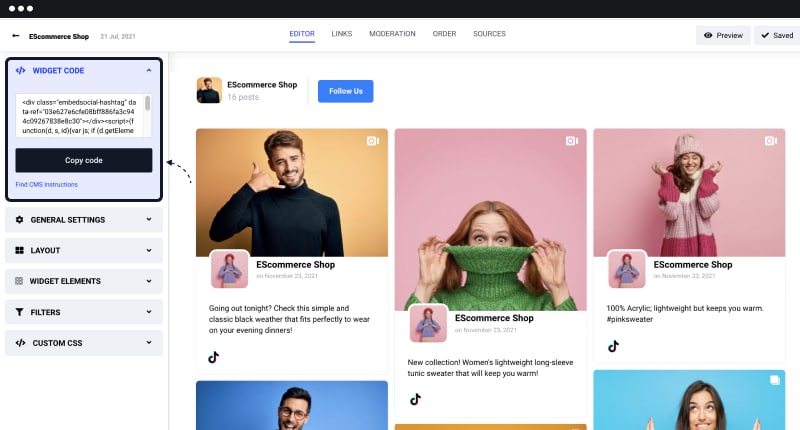**Detailed Caption:**

The screen capture depicts a detailed view of an e-commerce website interface, dated July 21, 2021. At the top, there is a thin black navigation bar featuring three white circles. Beneath it, a white banner with a gray underline displays "ES Commerce Shop" in bold black text, accompanied by the date "21st, July, 2021" in gray, with a black arrow indicating a dropdown next to the shop's name.

Below this banner, a series of clickable links are available: "Editor" highlighted in blue, followed by "Links," "Moderation," and "Order Sources" in gray. Adjacent to these, there are two functional buttons: a gray box labeled "Preview" with an eye icon, and another gray box labeled "Saved" with a check mark icon.

On the left side, a light blue box contains blue and black text reading "Widget Code," followed by a widget code for users to copy and paste. Visible nearby is a gray scroll bar. Moving towards the bottom, a black box with white text says "Copy Code," accompanied by a black arrow pointing to it. Below this, in blue text, is "Find CMS Instructions."

Further down, a series of gray and black pull-down menus include options such as "General Settings" with a cogwheel icon, "Layout" represented by small square icons, "Widget Elements," "Filters" with a funnel icon, and "Custom CSS," each entry flanked by arrows for navigation.

In the main white background body of the screen capture, several images with accompanying text are displayed. At the top, a square gold background showcases a Caucasian man with brown hair and facial hair, wearing a black turtleneck and posing with his hand in a telephone gesture. Next to this image is a blue box with white text instructing visitors to "Follow Us."

Beneath, a larger version of the same man's profile picture appears, with the site name "Yes, Commerce Shop" and an overlay of a white camera icon. Adjacent to this is a caption under a woman in a periwinkle long-sleeve shirt with braids, dated November 23, 2021. It reads: "Going Out Tonight? Check this simple and classic black weather that fits perfectly to wear on your evening dinners."

Following this, another image with a pink background features a redheaded woman in a green turtleneck pulled up over her nose and mouth, with a playful expression. The caption announces: "New collection: woman’s lightweight long sleeve tunic sweater that will keep you warm."

The next photo showcases a brunette woman wearing a dark pink and light pink sweater paired with a pink knit cap, with text stating: "100% acrylic lightweight but keeps you warm, #pinksweater."

Partially visible images at the bottom include a brown-haired man with glasses laughing, a segment of a gold bar, and a blue background featuring a brown-haired woman with her hands raised.